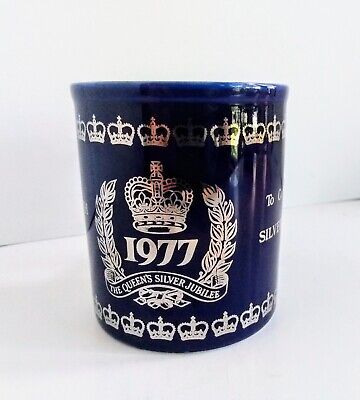This vertical, close-up crop of a navy blue shot glass showcases intricate and elegant detailing. The petite drinking vessel is adorned with a line of gold crowns encircling the top edge, mirrored by a similar row at its base. Dominating the center is a larger crown flanked by leaf laurels, with the year 1977 proudly displayed at its heart. Below this central motif, a banner proclaims "The Queen's Silver Jubilee." While the background is a plain white, lending contrast, the rich navy color of the glass itself stands out, emphasizing the classy and commemorative design. Along the right edge, partially obscured text includes the words "two" and "silver." The overall effect is one of regal elegance, befitting the occasion it celebrates.